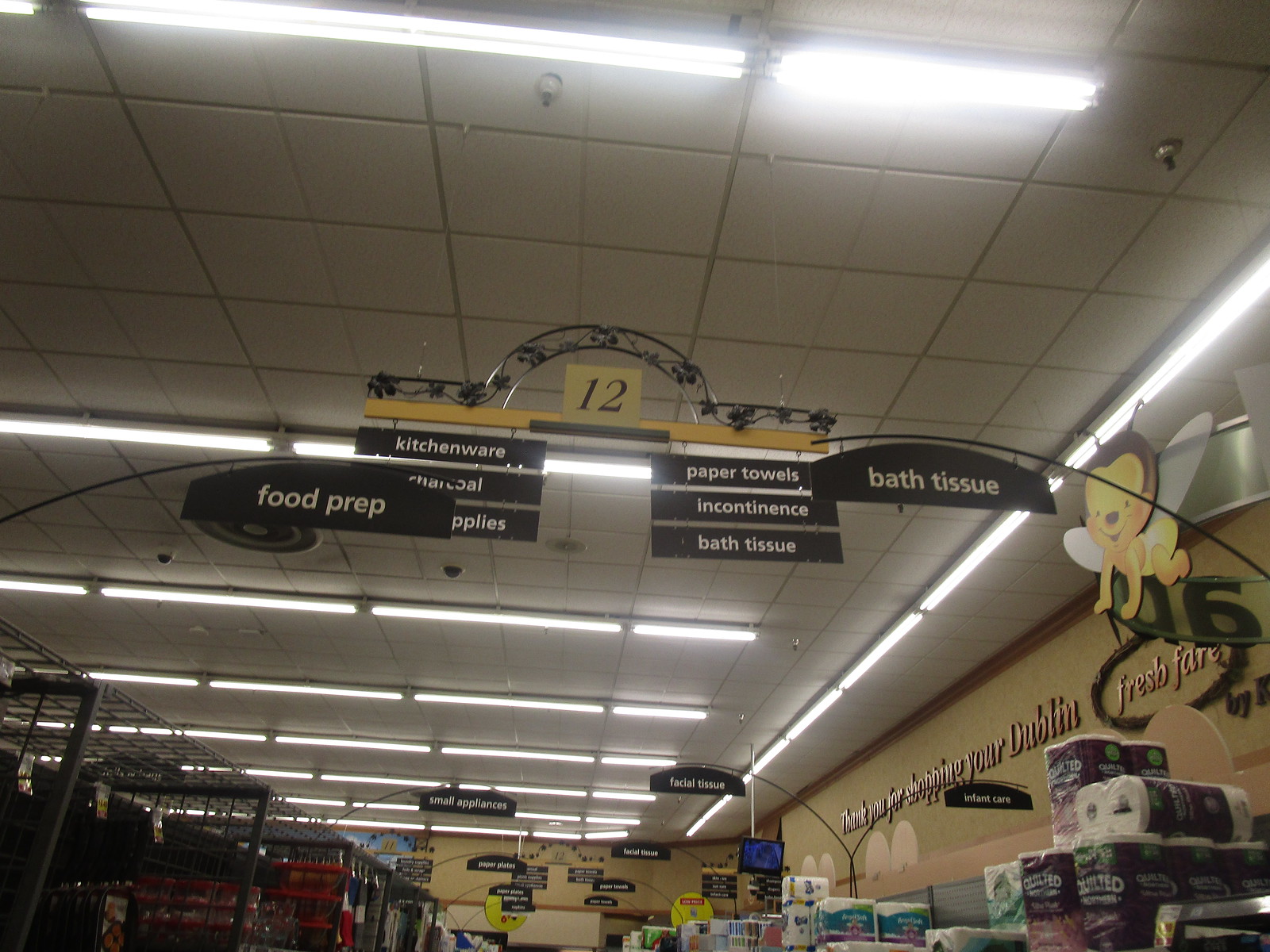This photograph captures the interior of a retail store from a floor-level perspective, looking upward. Dominating the view is a long, metal-framed sign that spans the entire aisle, adorned with a subtle floral pattern. The large number "12" is prominently displayed, accompanied by various item categories including "Food Prep," "Bath Tissue," "Paper Towels," "Incontinence," "Kitchenware," "Charcoal," and part of the word "Supplies."

Above, the white-tiled ceiling is lined with long, illuminated fluorescent lights. The wall is painted a pale cream color, providing a neutral backdrop to the scene. High on this wall, a welcoming message reads, "Thank you for shopping your Dublin Fresh Fare."

On the left side of the aisle, shelves laden with bathroom tissue can be seen, while various merchandise hangs from racks. Additional signs in a dark brown color are visible further down the aisle, guiding customers to different sections. On the upper right portion of the wall, near the ceiling, there's a whimsical cutout of a baby angel wearing a diaper, crawling and smiling, adding a charming touch to the store's decor.